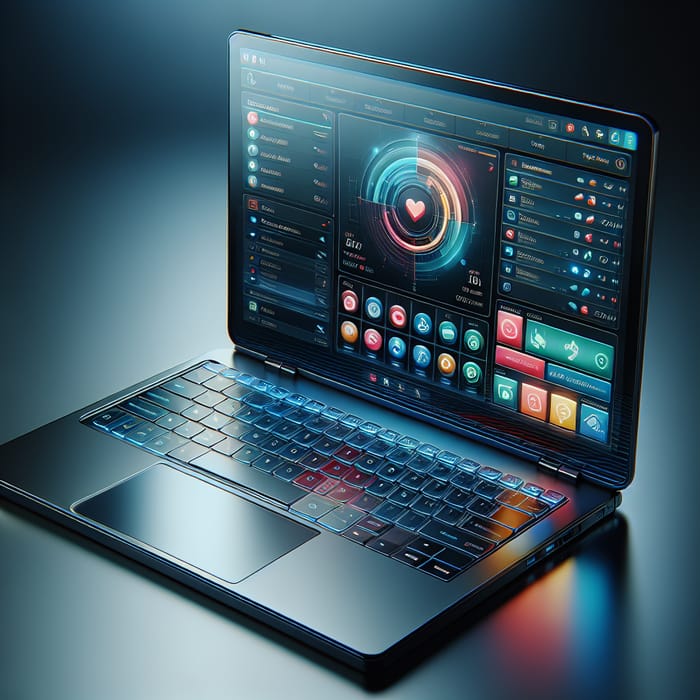This 3D rendered image depicts a square-shaped scene with equal dimensions on all sides, featuring a prominently placed black laptop. The laptop is open and angled towards the bottom left corner of the image, positioned on a glossy, reflective black surface within an otherwise featureless room. The laptop’s keyboard, which has blue light glowing from behind the white lettering, appears poorly rendered with many misshapen keys, suggesting an AI generation. Below the keys, a rectangular trackpad is visible. The laptop’s screen is displaying a complex graphic: a central heart encircled by a radial ring that transitions through red, blue, green, and yellow quadrants. Surrounding the main graphic are multiple icons and text, though the text remains illegible, reinforcing the artificial nature of the rendering. The backdrop transitions from a solid grey to a darker shade towards the top, adding to the overall mysterious and futuristic aesthetic of the image.